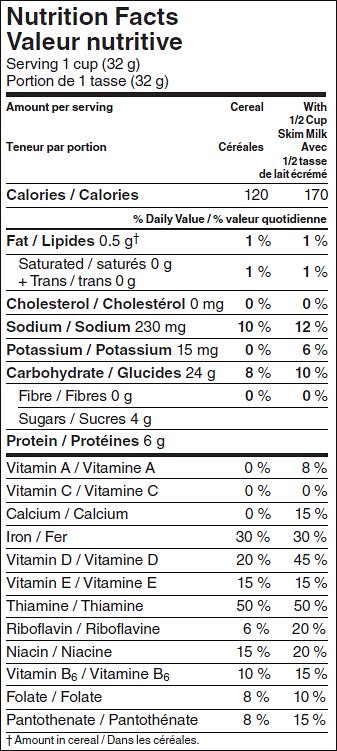The image is a screenshot of a Nutrition Facts label for a cereal, presented in both English and French. The label, encased in an upright white rectangle with black text, begins with the title "Nutrition Facts" followed by its French equivalent, "Valeur Nutritive." It specifies a serving size of one cup (32 grams), and includes detailed nutritional information for both the cereal alone and when combined with half a cup of skim milk.

The calories are listed as 120 for the cereal alone and 170 with milk. Fat content is 1 gram (1% daily value), with saturated fat also at 1% for both conditions. Cholesterol is 0 mg (0%), sodium is noted at 230 mg (10% alone, 12% with milk), and potassium is 15 mg (6%). Carbohydrates total 24 grams (8%), increasing to 10% with milk. Sugars are detailed as 0 grams (0%) for sucres, with a firm 4 grams for sugars. Protein content is 6 grams.

The vitamin and mineral section includes:
- Vitamin A, Vitamin C, calcium (0% solo, 8% with milk), iron (30%), Vitamin D (20%, 45% with milk), Vitamin E (15%, 50% with milk), thiamine (50%, Red Bull flavor), niacin (15%, 20% with milk), Vitamin B6 (10%, 15% with milk), folic acid (8%, 10%), and pentothenate (8%, 15%).

This comprehensive nutritional information is all presented in clear black lettering, making it easy to read and understand.